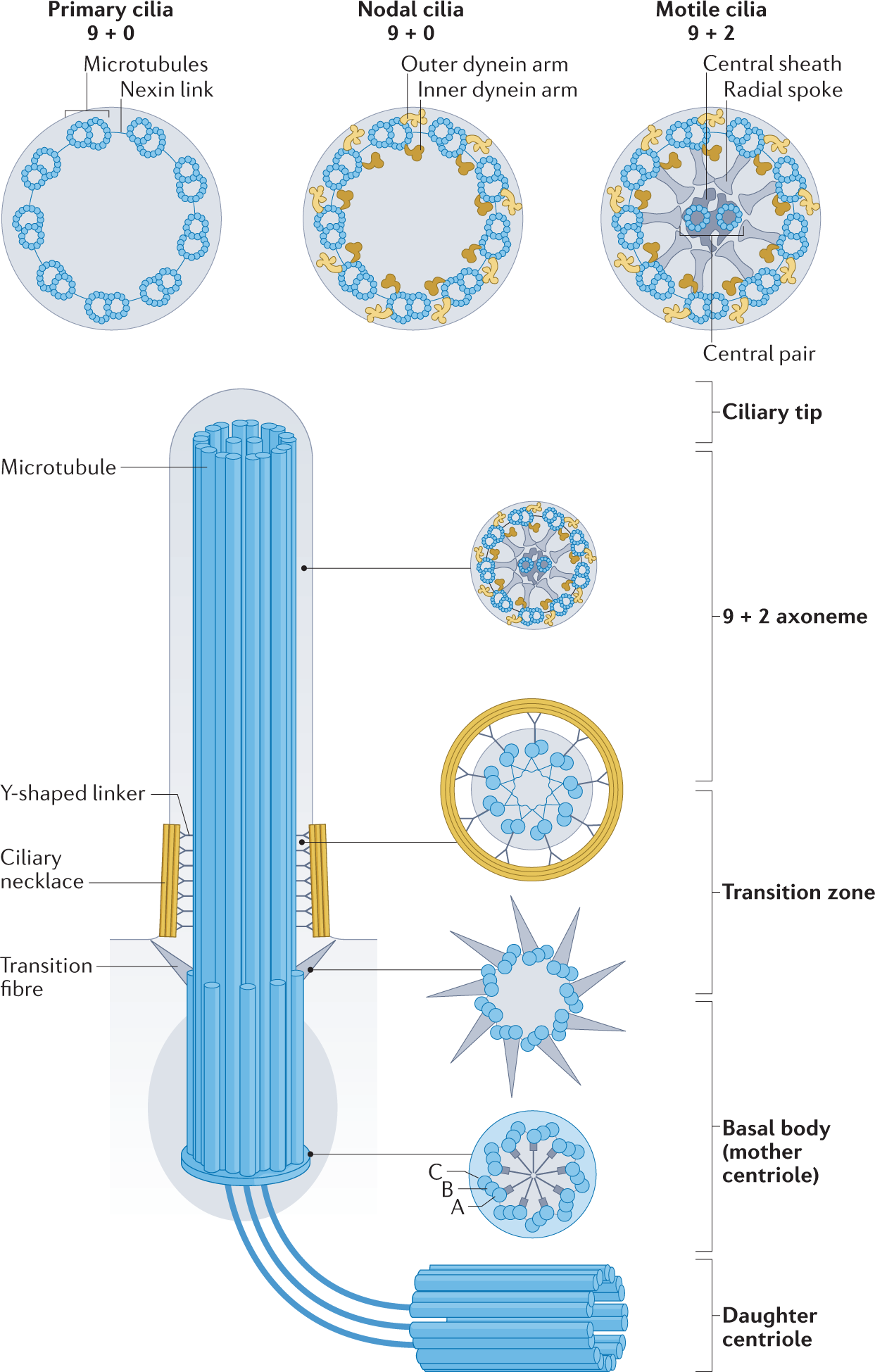The image is a detailed scientific illustration, resembling those found in biology textbooks, depicting various types of cilia and their structures. 

At the top of the diagram, there are three circular illustrations:
1. The first circle is labeled "Primary Cilia, 9+0," showing blue microtubules arranged in a figure-8 shape, connected by thin Nexin links.
2. The second circle is labeled "Nodal Cilia, 9+0," which, in addition to the features of Primary Cilia, has brown squiggles representing the outer dynein arms and yellowish squiggles for the inner dynein arms.
3. The third circle is labeled "Motile Cilia, 9+2," and includes a central pair of blue microtubules encased in a central sheath, with radial spokes (resembling wagon wheel spokes) stretching outwards and appearing as gray bone-like elements.

Below these circular illustrations is a detailed longitudinal section that appears like an elongated tube made of blue fibers, symbolizing a microtubule. This section includes multiple labels:
- "Ciliary Tip" with a 9+2 axoneme structure.
- "Transition Zone," indicating the region with ciliary necklaces and Y-shaped linkers.
- The "Basal Body," which includes labels for the mother centriole and daughter centriole at the bottom.

The entire diagram provides an exploded view of the ciliary structure, detailing the microtubule components and their associated parts, such as the central sheath, radial spokes, transition fibers, and ciliary necklaces.